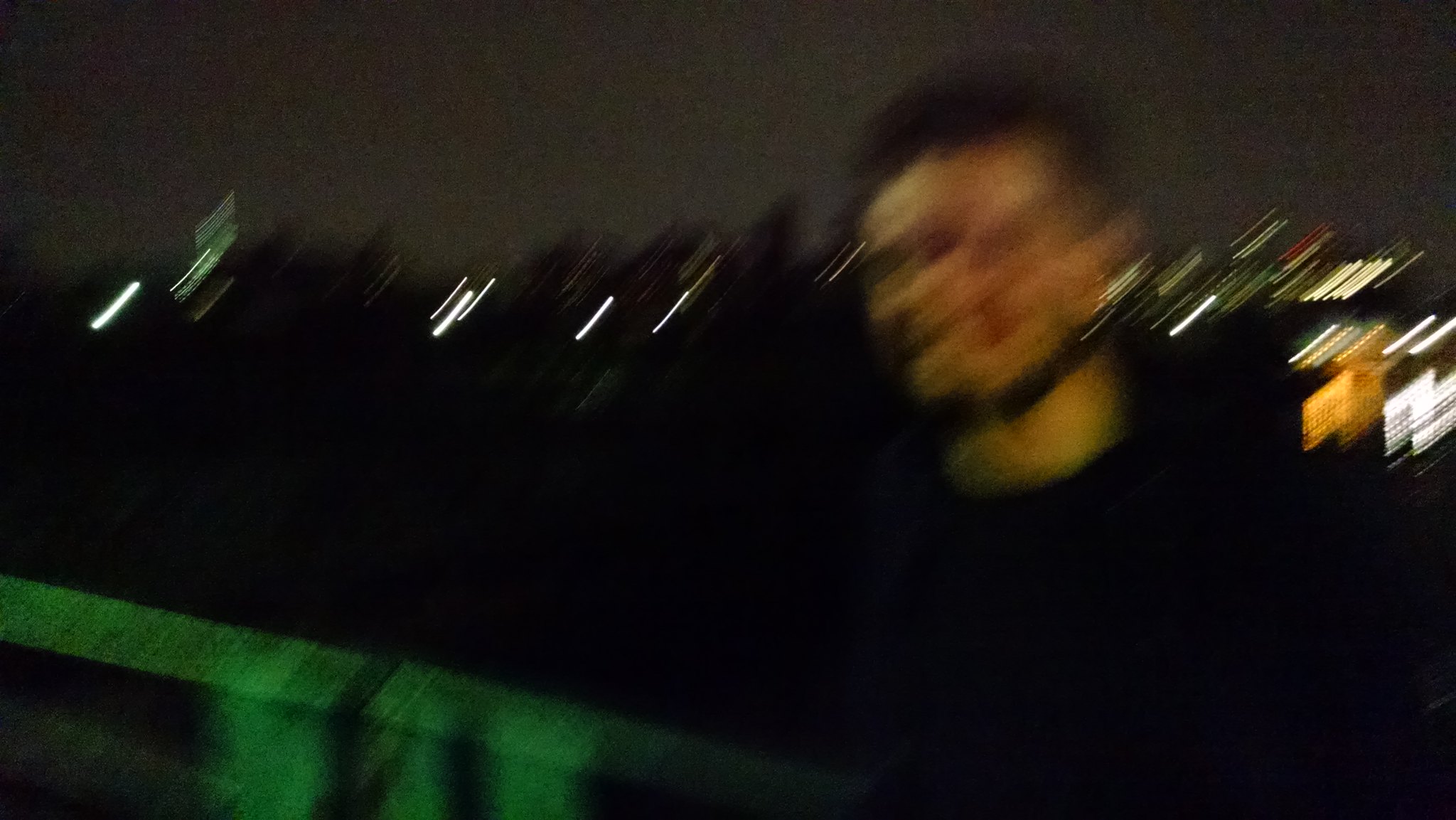This photograph, captured with a slow shutter speed at night, beautifully illustrates the essence of motion and time. In the foreground on the right, a man stands before a green-tinted retaining wall, but his face and form are artistically blurred, creating a ghostly appearance. The retaining wall extends into the middle ground, leading the viewer's eye deeper into the frame. Behind the man, the night sky paints a stark contrast, highlighted by streaks of light that are not of a cityscape, but rather the results of moving light sources. These lines of light sweep uniformly across the sky, indicating the camera’s deliberate vertical movement either up or down. This consistent blurring effect lends a dynamic rhythm to the image, encapsulating the ethereal beauty of both motion and stillness in one frame.